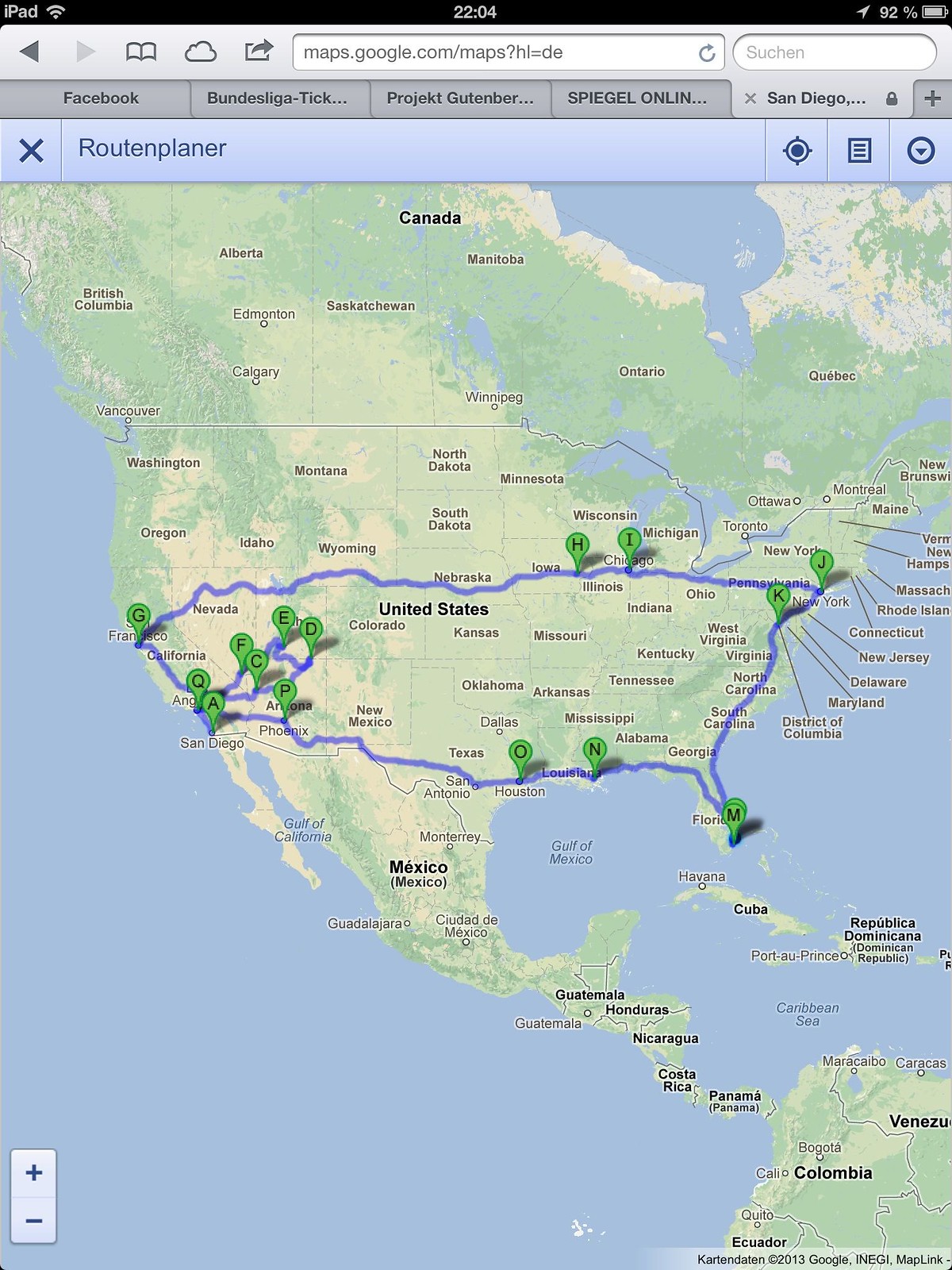Here is a detailed and cleaned-up descriptive caption:

"A screenshot taken from an older model iPad displays Google Maps in military time at 22:04, with the battery life at 92% and the location services active. The URL at the top reads maps.google.com/maps, indicating a search in English as reflected by 'search' in the search bar. The map spans North America, showing Canada, the United States, and Mexico. Various locations in the United States are marked with labels from A to Q, outlining potential routes for travel between multiple points throughout the country."